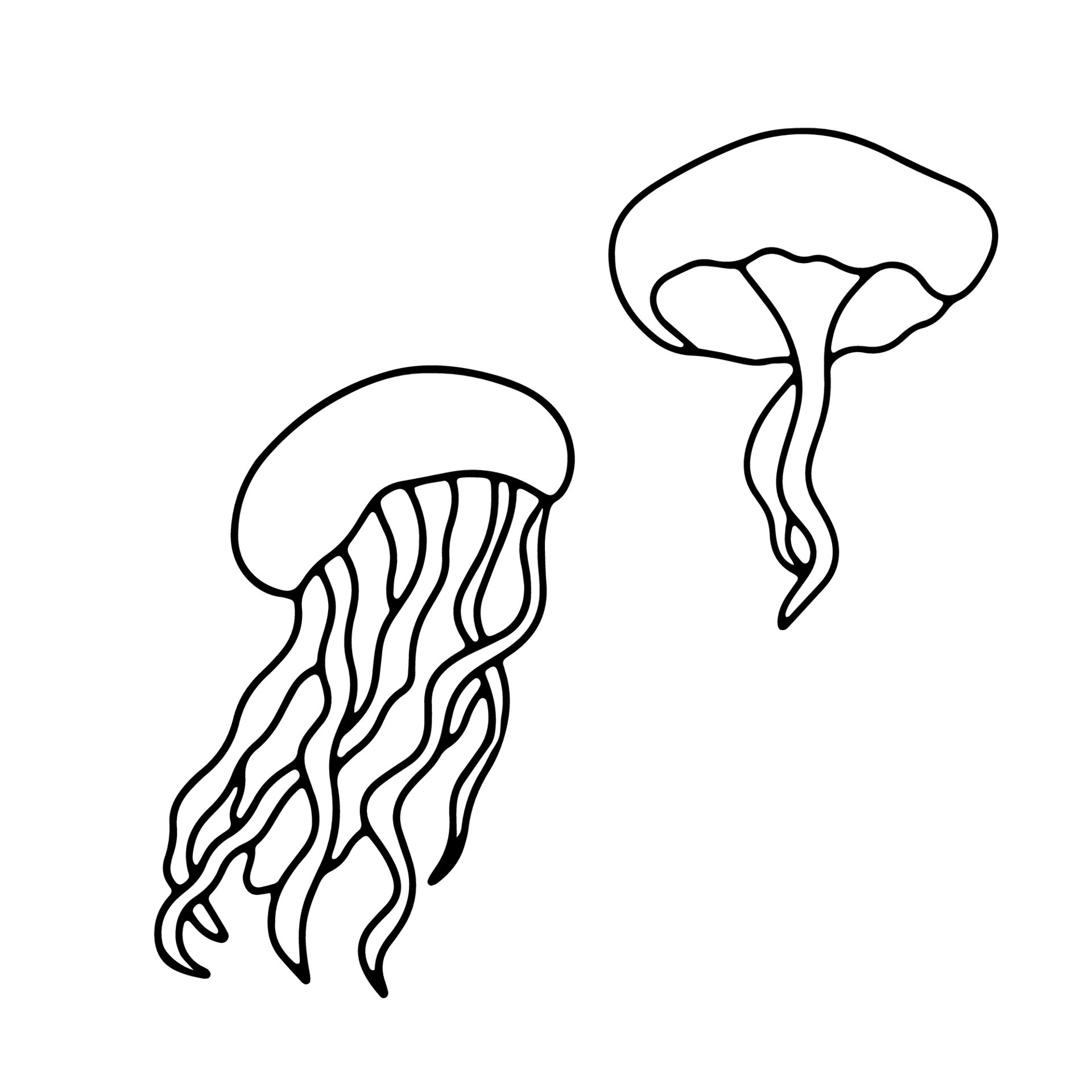The image depicts a simplistic, black and white line drawing on a white background, featuring two jellyfish. The top jellyfish, situated on the upper right, has a mushroom-like cap and two squiggly appendages extending downward, resembling legs. The bottom left jellyfish displays a similar mushroom-like top but with a greater number of appendages—approximately six to ten—streaming downward. Both jellyfish are rendered with fine black lines, creating an outline against the white interior and background, highlighting the stark yet elegant simplicity of the line art style.